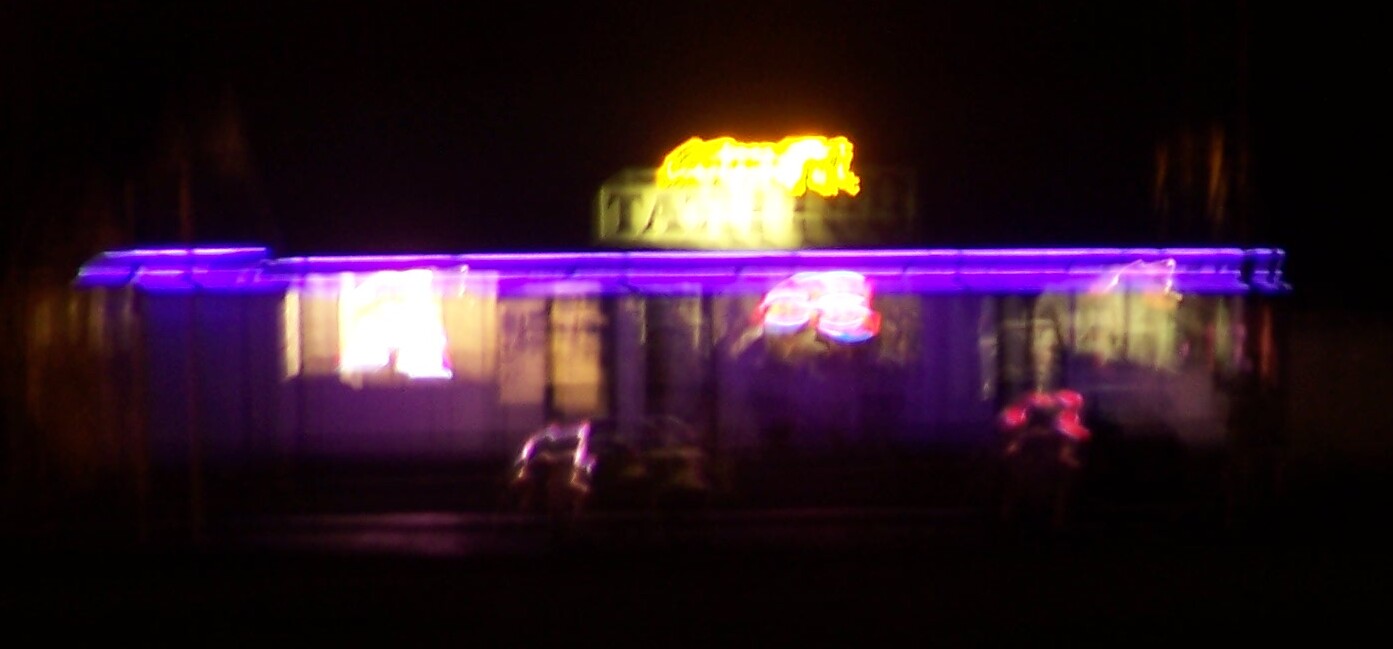In this photograph, we see a blurred night-time image of a diner or a diner-motel establishment, characterized by its distinct Southwestern architectural style featuring a low, flat roof. The forecourt of the establishment comprises a parking area directly in front of the building, where we observe the partial profiles and reflections of a few vehicles. The reflective surface of a curved vehicle roof is particularly noticeable amidst the blurred surroundings.

Illuminating the scene, blue neon trim adds a vivid, decorative touch along the structure, while the upper section of the photograph displays a sign with partially legible letters "TA", possibly suggesting the word "taco" or another form of advertisement. The brightness of the white neon lights has caused a double image effect, contributing to the overall blurred quality likely due to camera movement or a bump at the moment of capture. Dark skies envelop the background, intensifying the nighttime ambiance.

The windows of the building reflect more light and hint at an interior reminiscent of a classic diner, café, or potentially a motel. The entire aesthetic—marked by the building's design and layout, including a front parking area leading directly up to the entrance—evokes a quintessential Southwestern American roadside stop.